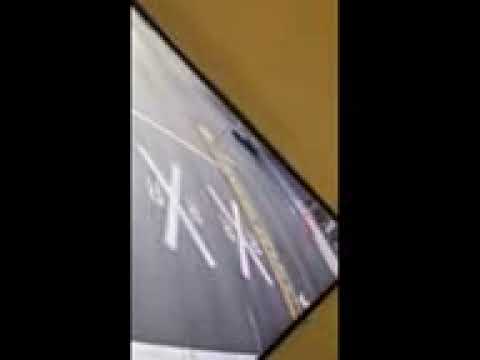The image is vertically oriented, featuring a central tan-brownish area resembling a wall, flanked on either side by solid black rectangular borders. At the heart of this image is a partially visible, rectangular section that seems to be part of a larger, cut-off scene. This central segment displays an asphalt road marked by faded white railroad crossing signs, including two X symbols with R letters, albeit upside down. The scene appears blurry or foggy, adding an element of mystery or wear and tear. Additionally, the image incorporates two brown triangles that frame the central scene. The overall composition suggests the remnants of a photograph or mirrored reflection, enclosed within a black frame, possibly a screen, that is slightly disjointed and cracked. The backdrop beyond this central rectangle is a solid mustard-yellow or dirt color, further contributing to the aged and ambiguous visual quality.